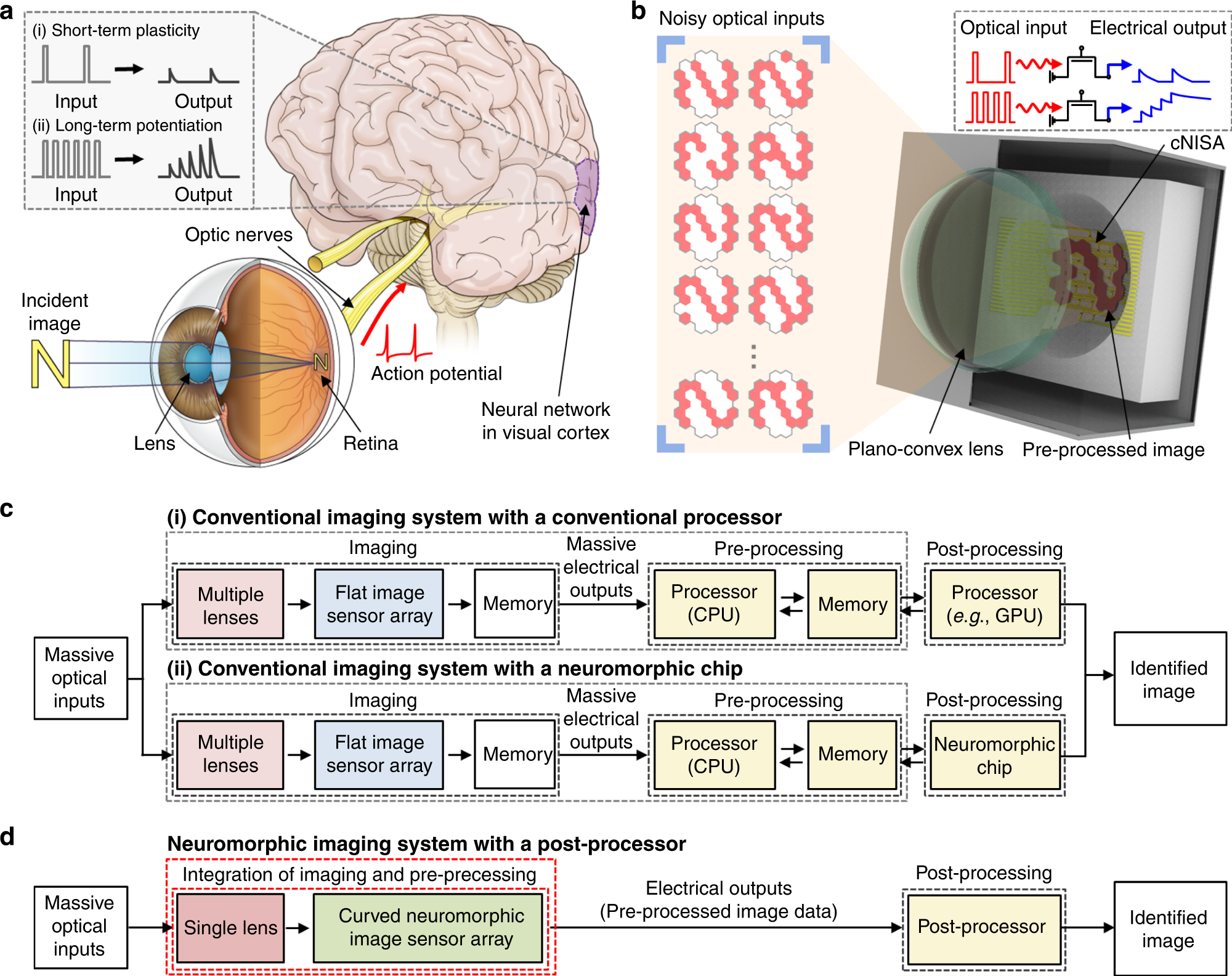The image is a highly detailed, scientific diagram divided into four sections labeled A, B, C, and D. Section A features a pinkish illustration of a human brain, highlighting the optic nerves and their connection to the visual cortex. It includes a close-up of an eye showing the lens and retina, with text discussing input and output related to the optic nerves' action potentials within a neural network. Section B depicts a diagram of a device with a plano-convex lens and labels the pre-processed and processed images; it explains the conversion of optical inputs to electrical outputs. Sections C and D contain complex flow charts and graphs, reminiscent of electrical schematics, detailing conventional and neuromorphic imaging systems' inputs and outputs with different processors. These sections emphasize massive optical inputs and how they are processed into identified images, illustrated with various colored text boxes and lines.